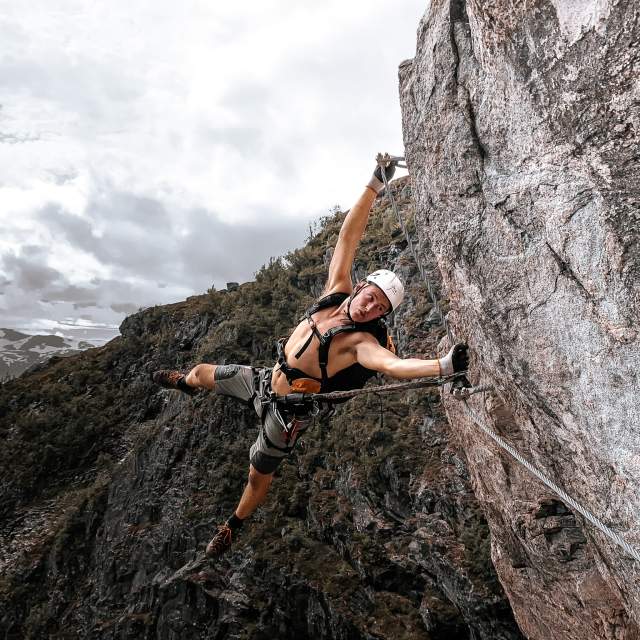This image captures a rock climber in the midst of a challenging ascent. The climber, a shirtless man, wears gray shorts and black ankle socks paired with brown climbing shoes. His hands are protected by gloves, and a white helmet shields his head. A black backpack with straps and a waist harness is secured to his body. He is gripping a steel cable that is anchored into the vertical, craggy gray rock face. The man is splayed out with one arm extended upward holding onto a hook, and the other arm positioned lower, also grasping a hook. His climbing gear includes a rope tied to his waist, adding extra security. The scene is set against a backdrop of gray skies filled with clouds and the rock face, which exhibits patches of dark green vegetation. The image appears to be edited for a slightly reddish-gray tone, enhancing the dramatic atmosphere of the climb.